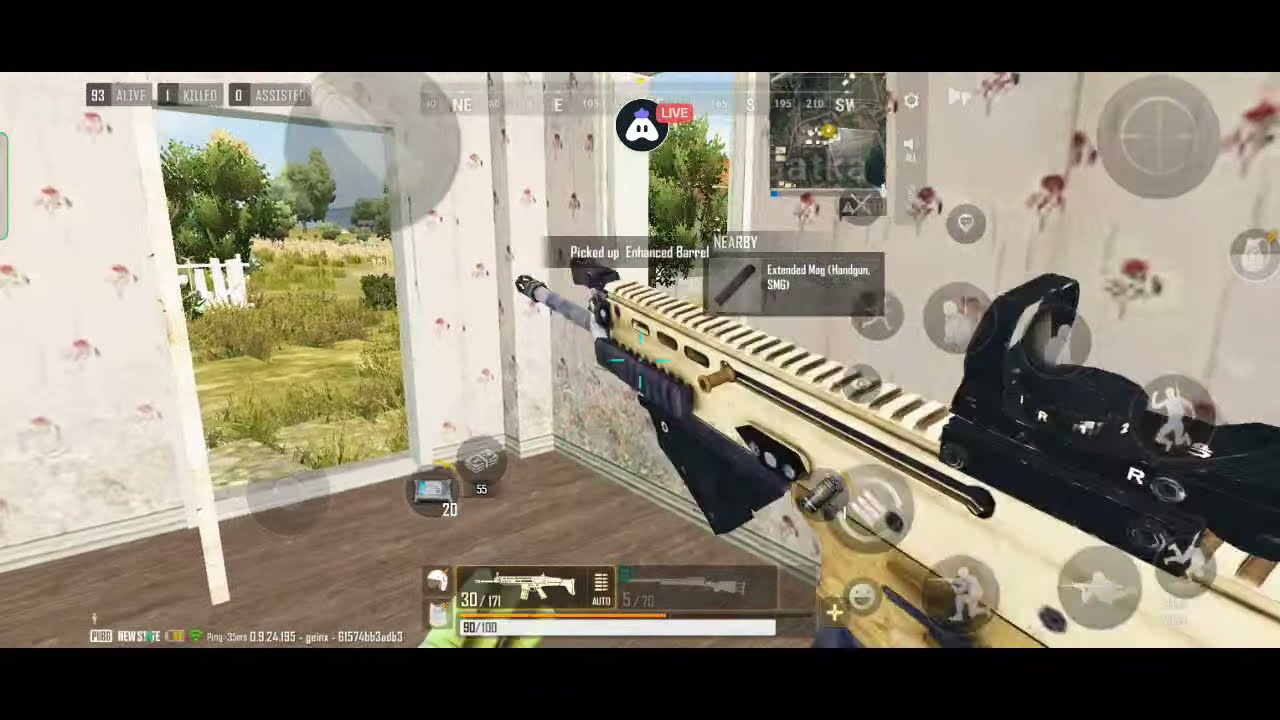This detailed screenshot from a video game, possibly PUBG or a similar title, captures the immersive scene inside a room. Dominating the right side of the image, an automatic rifle, cream and black in color, extends toward the upper left. The rifle features a black tip, grey barrel, a black scope, and a distinct brown knob with two slits, along with three rectangular holes aligned in a row. A bolt extends an inch from the left side of the gun. The room's walls are adorned with white wallpaper accented by red roses with green stems and leaves. The brown floor has variations in color adding depth to the setting. To the left, an open door reveals an outside area with grass, stones, a dilapidated white picket fence, trees, and a glimpse of the sky. Additionally, a window on one of the walls allows another view of the outdoor scenery, showcasing more trees and sky. The bottom middle of the screen displays a list of weapon options, while the top left corner features game stats. The top middle of the screen includes a map and additional text, adding to the game's comprehensive HUD.